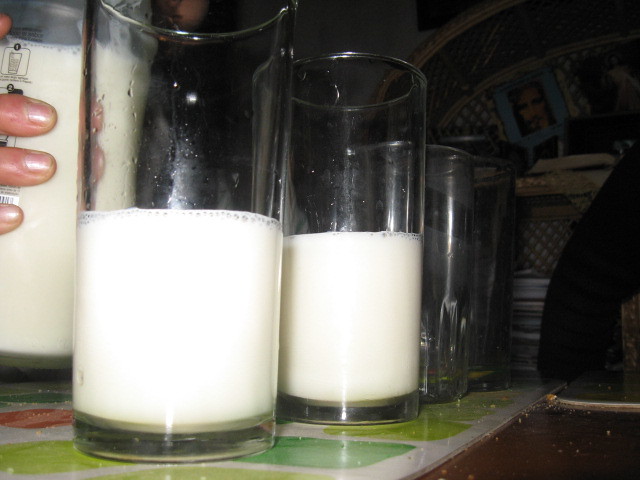This close-up color photograph, taken at countertop level, captures a row of four clear cylindrical glasses on a white counter adorned with green and red patterns, resembling a restaurant tabletop. The two glasses on the left are half-filled with a white liquid, likely milk, with visible bubbles near the top. The remaining two glasses to the right appear empty against the dark background. On the far left side of the frame, three fingertips with pearl-colored nail polish hold a nearly full bottle of the same white liquid, suggesting milk. The tabletop extends left with a white patterned placemat overlaying a brown surface.